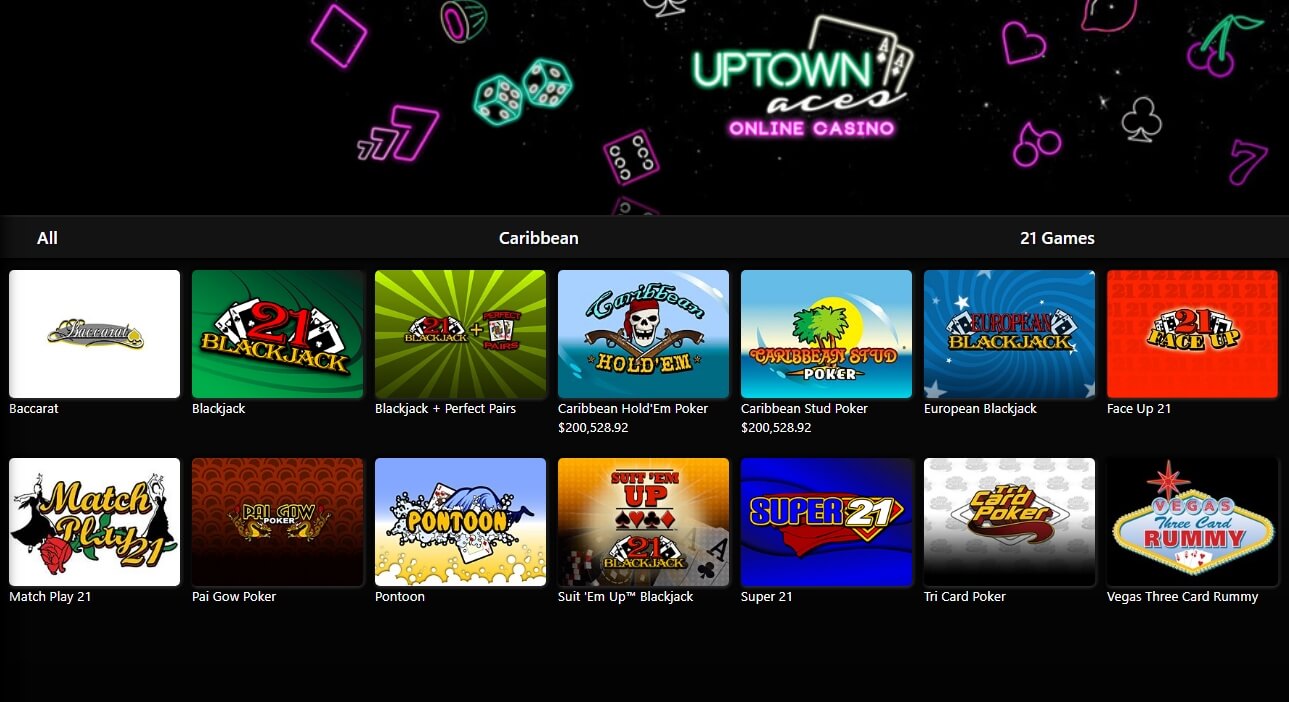The image features a dynamic and visually engaging layout on a black background. At the top, there are several vibrant visuals including a purple diamond, teal-colored dice, and purple-colored dice. Below these, the text "Uptown Aces" is prominently displayed, enhanced by an overlay of two ace poker cards, adding a touch of classic casino imagery.

Directly beneath, the phrase "Online Casino" is boldly presented in a vibrant, neon purple font, accompanied by an assortment of colorful icons: a purple heart, purple cherries, a purple clover, a purple and green cherry symbol, and a purple seven, all contributing to the playful and energetic theme.

Following this, a dark gray menu bar is outlined, displaying the options "All Caribbean" and "21 games." Below the menu, there are two horizontal rows, each comprising seven different game thumbnails. In the top row, the second thumbnail from the left stands out with a green background and the text "21 Blackjack." Another notable thumbnail, two places to the right, showcases a skull and crossbones with crossed guns, labeled "Caribbean Hold'em." Adjacent to this, the next thumbnail features the title "Caribbean Stud Poker," rounding out the display with a sense of variety and excitement.